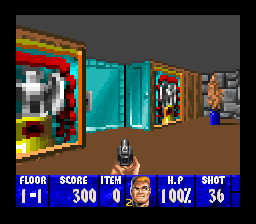This image is a still frame from an early 90s first-person shooter video game, likely from the era of Doom or Duke Nukem. The screen displays an underground room filled with pixelated, 8-bit graphics. At the bottom of the screen is a blue heads-up display (HUD) bar featuring various game statistics: "Floor 1-1," "Score 300," "Item 0," "HP 100%," and "Shot 36." The HUD also includes the player's character avatar, depicting a craggy-faced, short-blonde-haired man with the number "2" beside it. 

The player's view, from a first-person perspective, shows a pair of hands holding a grayish-black gun. In the room, there are several distinct elements: a large metal door, a green door, a blue door at the center, and a narrower door off to the right. In the background, part of the stone wall is visible on the upper right. Near this area, there's a non-playable character (NPC) wearing a khaki trench coat and blue pants, standing idly with short black hair. The walls and pathways depicted are navigable, with some blurred imagery, adding to the classic, retro gaming aesthetic.